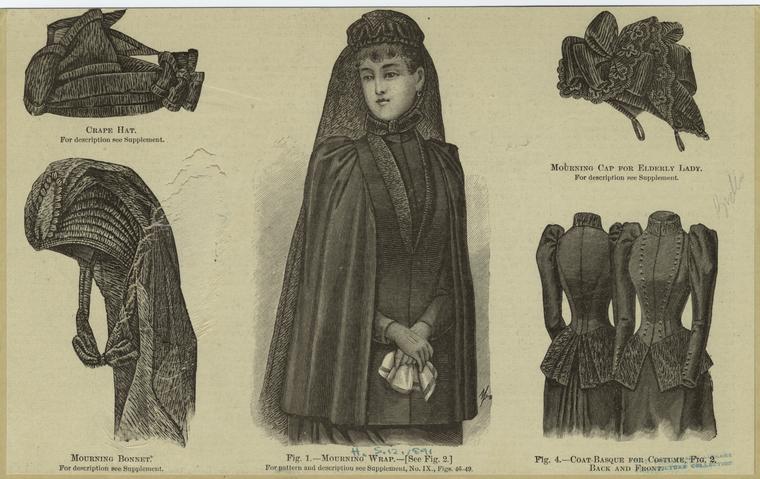The image is an old newspaper or magazine clipping with a yellowed, parchment-like appearance and various shaded illustrations in black, white, and gray tones. Dominating the center is a large illustration of a woman, resembling a figure of royalty, wearing a formal mourning wrap and holding a handkerchief. She has a veil tied around her head. The illustration is labeled "Figure 1, Morning Wrap" with a note to "see figure two for pattern and description" and to "see supplement number five or six."

On the left side, there's a "Crape Hat" at the top and a "Morning Bonnet" below it. The right side features a "Morning Cap for Elderly Lady" in the top corner and another illustration labeled "Figure 4, Coat Basque for Costume" in the bottom corner. The layout includes five illustrations, each with descriptive text labels, suggesting a focus on mourning attire and related accessories, all presented in a grayscale palette that adds to the vintage feel of the clipping.